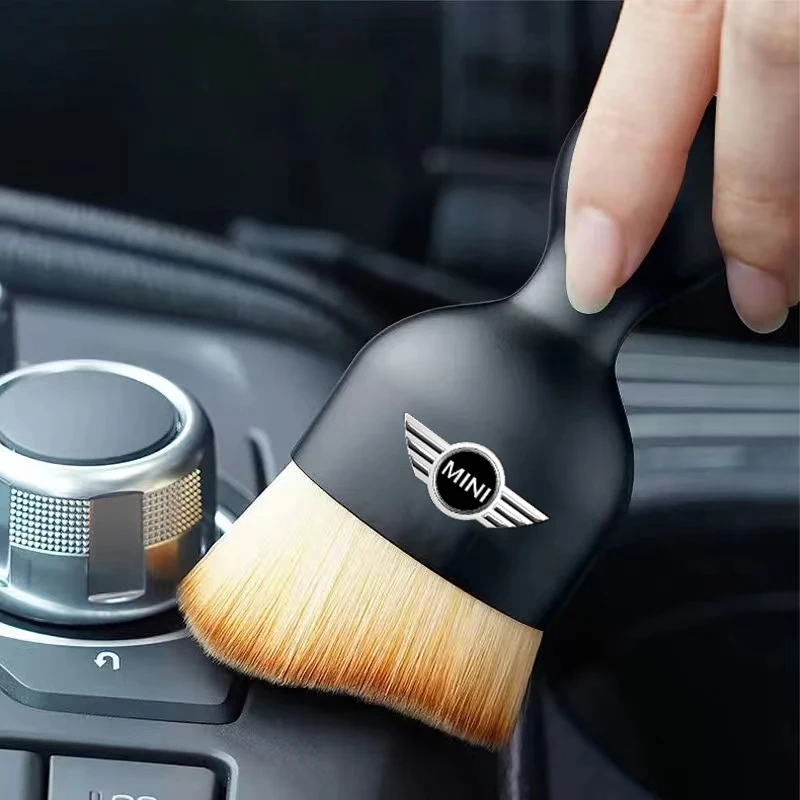The image depicts a detailed close-up of a car's center console, likely belonging to a MINI Cooper, given the prominent branding. The central focus is a black-handled brush held by what appears to be a woman's well-manicured hand, with the index and middle fingers visible and bearing long, unpainted nails. The brush handle features the MINI logo, characterized by the word "MINI" in silver uppercase letters within a black circle, flanked by silver wings outlined in black. The bristles of the brush exhibit an ombre effect, transitioning from light beige at the base to a burnt orange-reddish hue at the tips. The brush is actively sweeping the black surface of the console near a distinctive round, silver control knob situated to the lower left, hinting at its function as a cleaning tool. The image captures the texture and subtle details of both the brush and the car's interior, set against a backdrop of smooth, dark surfaces and partially visible buttons, conveying a meticulous scene of car care.